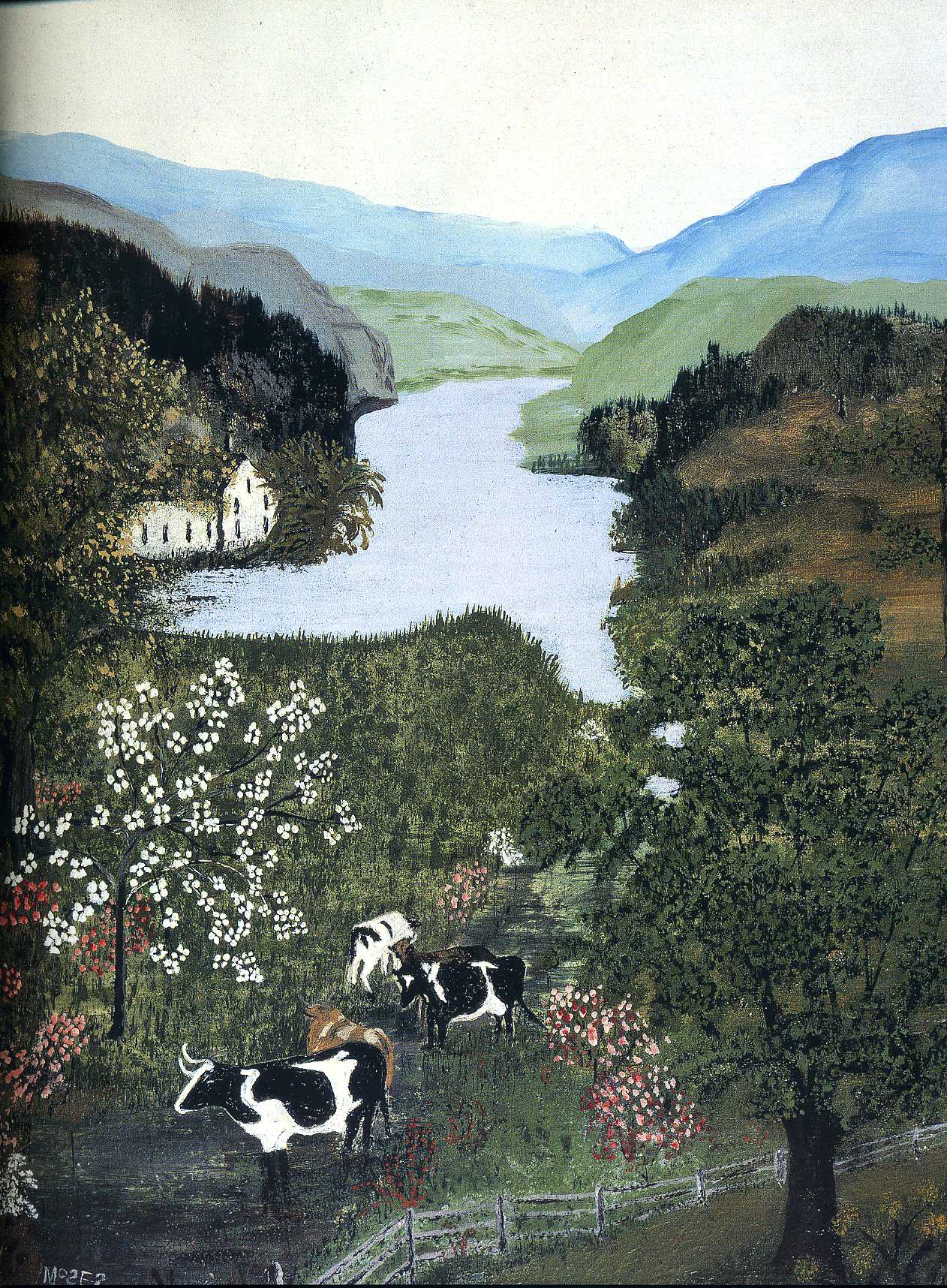This vivid painting showcases a serene natural landscape in portrait orientation, featuring a lush green pasture where four cows—three black and white, and one brown and white—graze peacefully. The lower area of the painting depicts a charming rural scene with green grass, blooming trees adorned with white and red flowers, and colorful floral bushes. A white wooden picket fence stretches from the bottom center towards the upper right.

In the middle ground, there is an H-shaped blue water body, likely a lake or river, with the left side partially obscured by trees and the hint of a house whose white walls and black rectangular windows peek through the foliage. Further beyond the water, light green, light purple, and light blue mountains rise gently, creating a layered effect with the tallest peaks on either edge of the canvas. Crowning the scene, an off-white, bone-colored sky completes the tranquil ambiance. 

The painting is signed in the lower left-hand corner with what appears to be "M02F2," hinting at the artist's identification or a creative pseudonym. Overall, the artwork brilliantly captures the vibrant and peaceful essence of a countryside valley, possibly executed with oil paints, showcasing exquisite attention to detail and color.